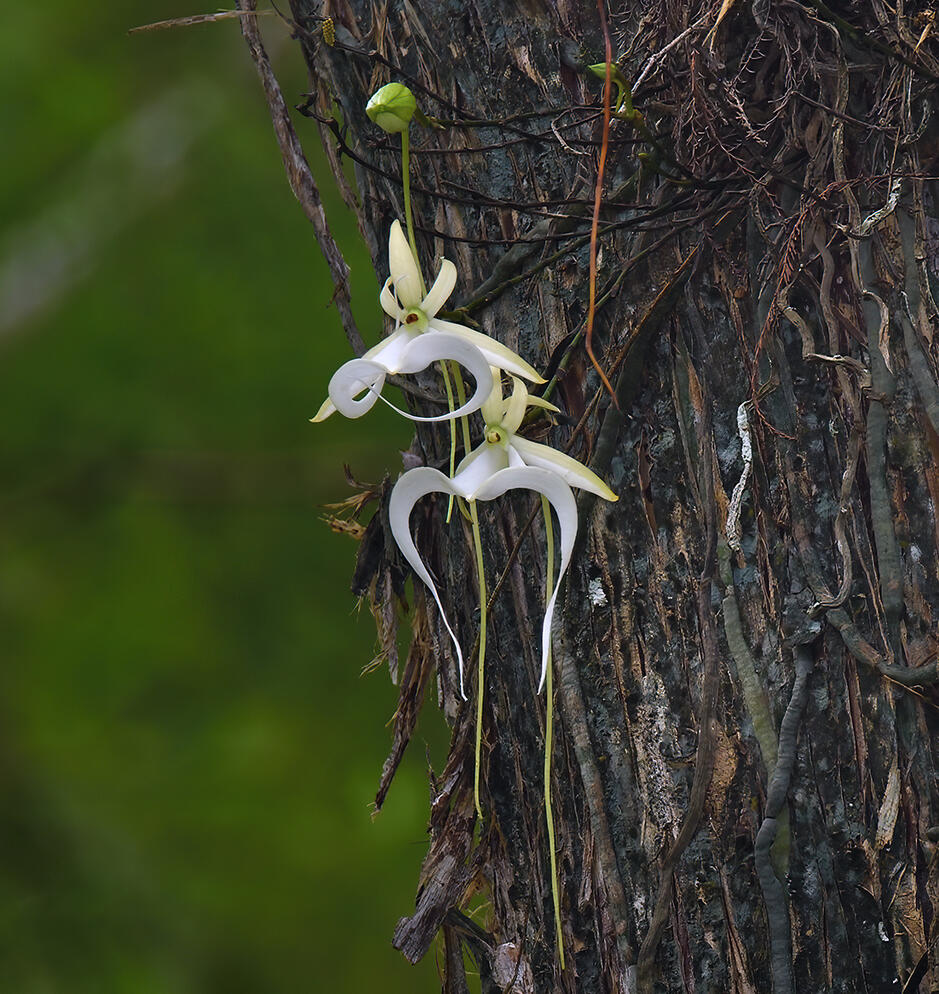The daytime photograph captures a scene of intricate natural beauty, albeit with a slightly surreal touch. Dominating the right-hand side of the image is a grayish tree trunk, heavily entwined with vines that appear tightly bound and somewhat wilted, yet adding an intriguingly textured look. There are numerous small green buds along these vines, hinting at new life. Notably, on the left-hand side of the tree trunk, two striking white flowers are in bloom, resembling orchids, with long, narrow petals that curl and curve in unusual, elaborate shapes. These petals have a subtle yellow tint at their base, enhancing their delicate appearance. The background of the image, slightly blurred, reveals shades of green and brown, reminiscent of leafy branches, contributing to the lush, natural atmosphere. The overall impression is of a strikingly beautiful, albeit strangely otherworldly, moment in nature.